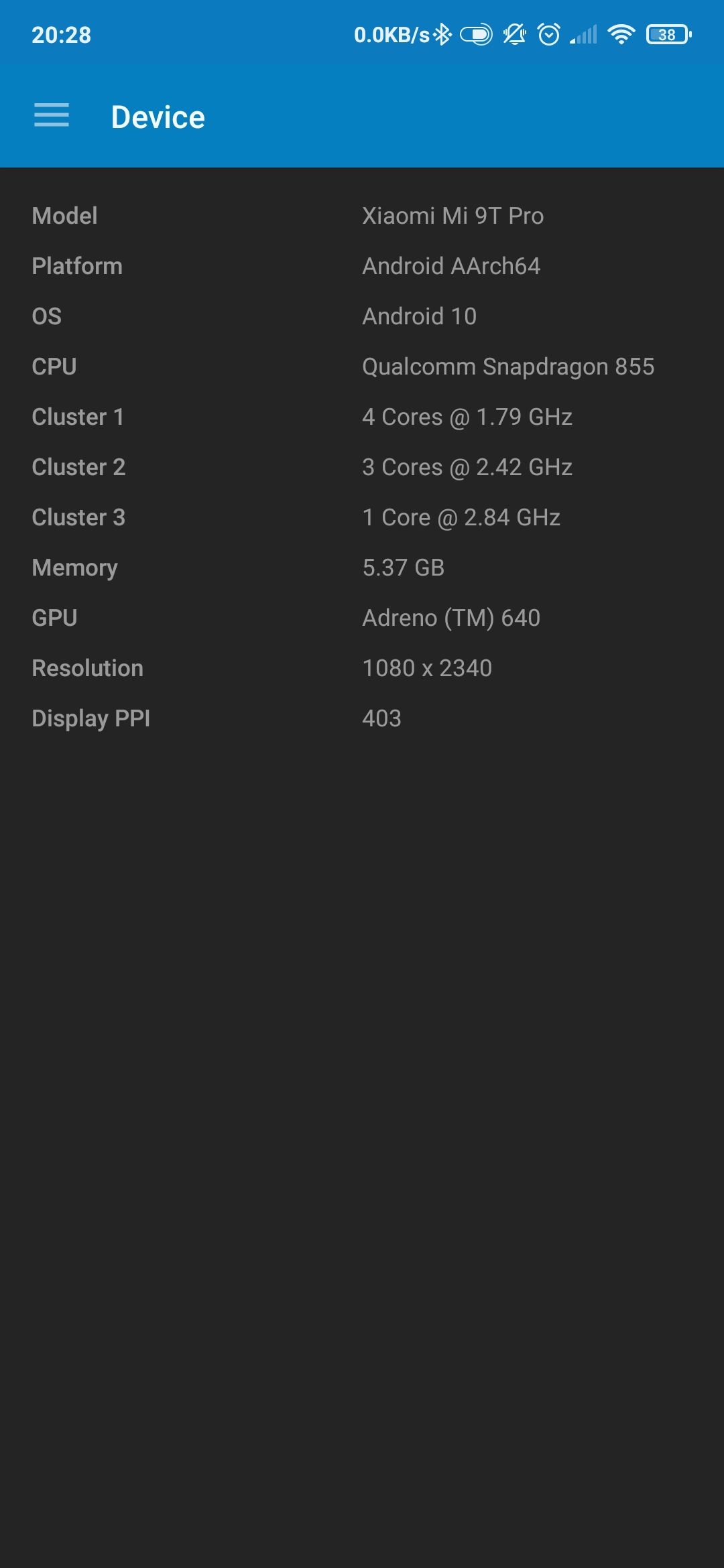This image, captured from a cell phone screen, features a detailed snapshot of the device's system information. At the top of the screen, the time is displayed as 20:28, flanked by various status icons such as the battery icon showing 38% remaining, Wi-Fi signal strength, and a clock, among others. In white text at the top, the word "Device" is prominently displayed next to three horizontal lines, suggesting a menu icon.

The screen's background is black, providing a high contrast for the white and colored text in the foreground. On the left side, two columns of detailed technical specifications are listed:

- **Model:** xx a commie mi NT Pro
- **Platform:** Android arch 64
- **OS:** Android 10
- **CPU:** qualcomm Snapdragon 855
  - *Cluster 1:* 4 cores at 1.79 GHz
  - *Cluster 2 and Cluster 3:* (contents not fully visible in the provided information)
- **Memory:** (details not fully visible)
- **GPU:** (details not fully visible)
- **Resolution:** (details not fully visible)
- **Display PPI:** PPI (with "PPI" capitalized)

The comprehensive breakdown of the device specifications, layout, and iconography provides a thorough insight into this cell phone's technical details.